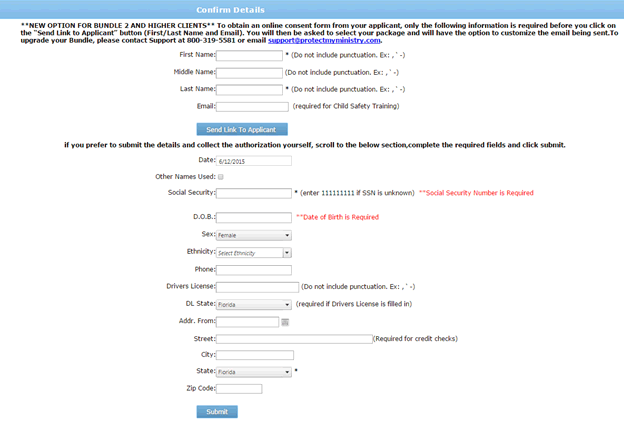The image showcases a webpage interface that facilitates obtaining online consent forms from applicants. At the top, a prominent blue bar features the text "Confirm Details" in white. Beneath this, it introduces a "New Option for Bundle 2," allowing clients to request online consent forms from applicants more efficiently. 

The necessary information to send the link includes the applicant's first name, last name, and email address. Users are then prompted to select a package and given the option to customize the email sent to applicants for upgraded bundles. For further assistance, clients are directed to contact support at 800-319-5581 or via email at support@protectmyministry.com.

The next section has fields for the applicant's first name, middle name, last name, and email, with notes next to some fields advising users not to include punctuation. A specific note mentions that the email is required for child safety training. A blue button labeled "Send Link to Applicant" enables users to proceed.

Additionally, there's an option for those preferring to collect authorization details manually. Instructions guide users to scroll to a below section, complete the required fields, and click "Submit." The required fields include details such as date, other names used, social security number, date of birth, sex, ethnicity, phone number, driver's license, state, street, city, state, and zip code.

Overall, the webpage has a white background with various text fields and instructions, highlighted by blue buttons with white text for navigation.